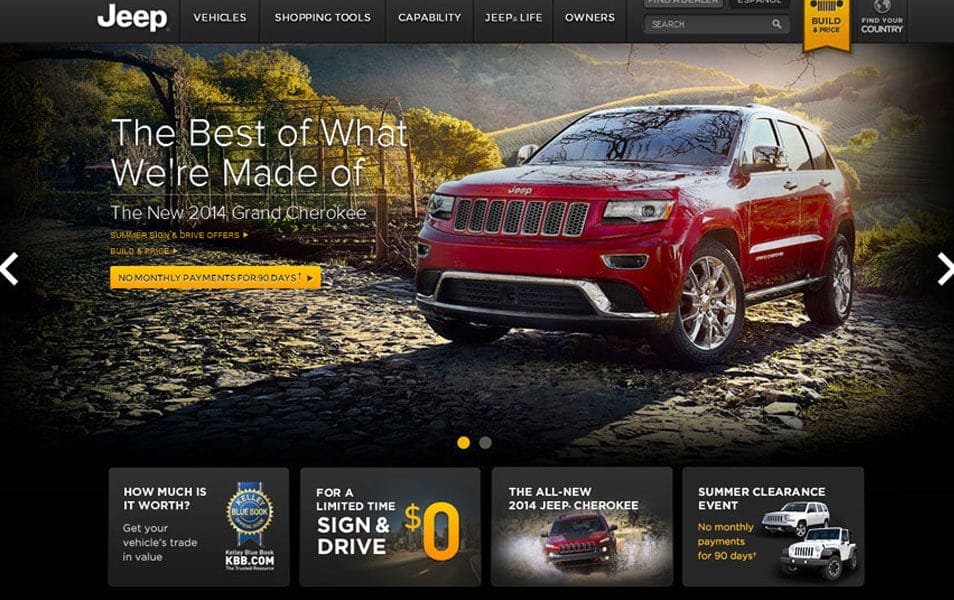**Caption: Screenshot of Jeep Website**

This screenshot captures the homepage of the Jeep website. In the upper left corner, the word "Jeep" is prominently displayed. To its right, there are several navigation sections: "Vehicles," "Shopping Tools," "Capability," "Jeep and Life," and "Owners." A search bar labeled "Search" with a magnifying glass icon is positioned to the right of these sections. Further to the right is a yellow "Build & Price" bookmark, followed by a "Find Your Country" button.

Beneath the navigation menu is a detailed banner featuring a vibrant image of a red Jeep SUV. The Jeep is shown on a gravel or stone path, with a picturesque backdrop of mountain ranges under a radiant sunrise or sunset. To the left of the image is bold text reading, "The best of what we're made of," accompanied by the subtitle, "The new 2014 Grand Cherokee." Below, yellow text promotes "Summer Slow and Drive Offers," with a clickable button advertising "No monthly payments for 90 days." Navigation arrows on the left and right sides of the banner indicate the ability to cycle through various banner options.

Below the banner are additional promotional sections. The first section offers a tool to determine the trade-in value of a vehicle, marked by a blue ribbon with "KBB.com" branding. To the right, another promotion highlights "For a limited time, Sign and Drive - $0," with "$0" emphasized in yellow. Adjacent to this is an image of the all-new 2014 Jeep Cherokee driving through water. Finally, on the rightmost side, a section titled "Summer Clearance Event" features two white Jeeps with yellow text announcing "No monthly payments for 90 days."